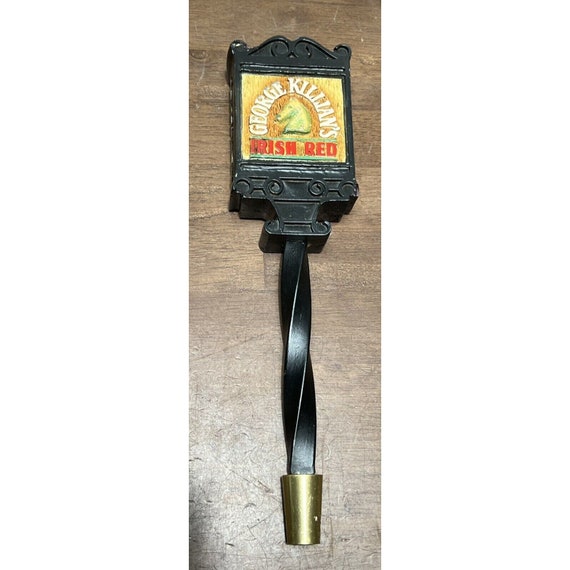This photograph captures a vintage beer tap handle, intricately designed and likely used in a bar setting. The handle rests on a distressed brown wooden surface and features a rectangular placard at the top. This placard showcases the branding for "George Killian's Irish Red," with "George Killian's" written in white and "Irish Red" in red. Central to this design is a prominent horse's head set against a yellow background, with the text partially arching around it. Extending from the placard is a long, twisted black iron stem, emphasizing craftsmanship and durability. The handle's base culminates in a shiny gold-colored tip, resembling a cork but made of metal. The overall structure and ornate details suggest its use as a decorative and functional lever for dispensing beer.